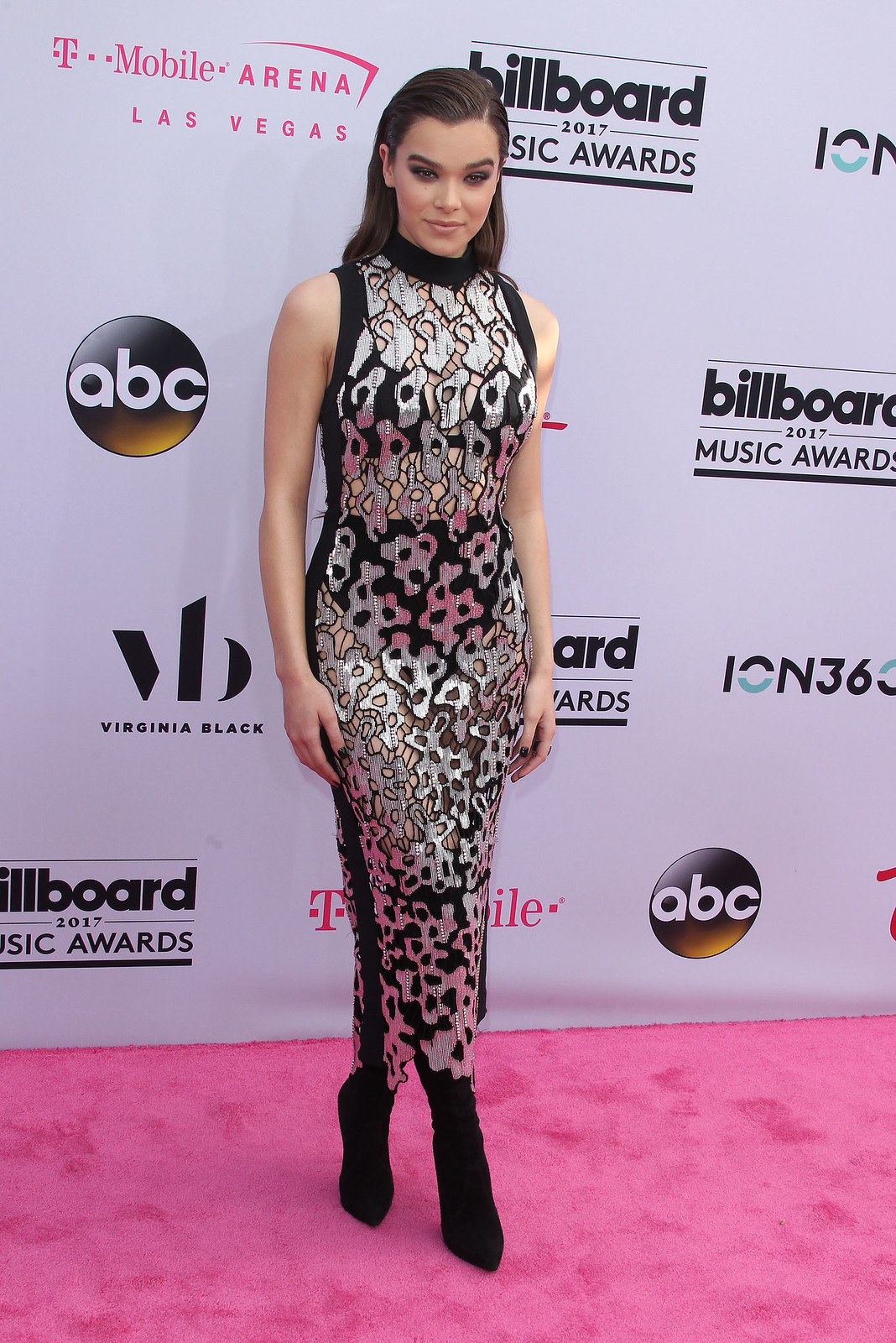The image features a woman, likely a celebrity, posing at what appears to be the Billboard 2017 Music Awards red carpet event. She is wearing a striking black and white shimmering dress, which has a somewhat transparent quality to it. The dress is sleeveless and paired with black stockings and black boots, showcasing her stylish attire. Her hair is slicked back and parted to the side, and she is adorned with bold eye makeup. The woman also has black nail polish, further complementing her sophisticated look. She is standing on a pink-colored carpet with her legs crossed, and gazing downwards at the camera. The backdrop behind her is white, adorned with multiple logos including T-Mobile Arena, Las Vegas, ABC, Virginia Black, and Billboard Music Awards, indicating the prestigious nature of the event.